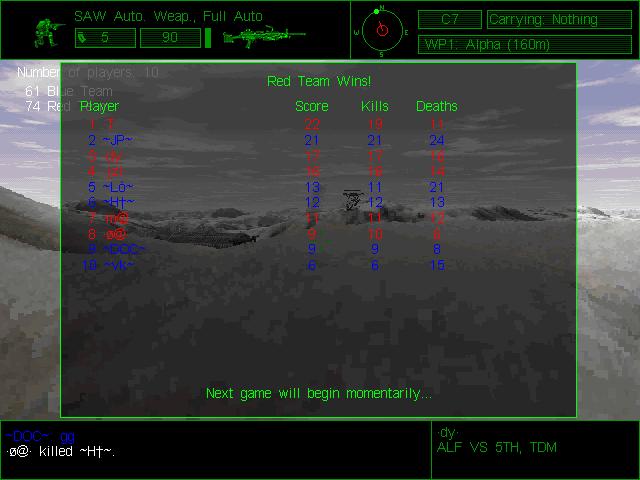This is a detailed screenshot of an old, pixelated military video game. The main highlight of the image is a prominent, gray rectangular box with a bright green digitalized outline occupying the center. This box displays a leaderboard, indicating that the "Red Team Wins." Beneath this heading, there are four columns labeled "Player," "Score," "Kills," and "Deaths." The player names, written in Asian script, and their corresponding statistics are displayed in ten lines. The scores and stats are mostly two-digit numbers, with half of them in red and the other half in blue. A green text at the bottom announces, "Next game will begin momentarily."

The image also features a black border on both the top and bottom. In the top left corner, there is a pixelated green figure of a soldier kneeling on one knee, pointing a gun, identified by stats next to him that include labels like "saw," "auto," and "wep." The gun image also appears next to these stats. The upper right corner of the image showcases a green compass symbol indicating north, south, east, and west, and displays coordinates like "WP1 alpha (160 meters)." In the bottom left corner, white text stands out with an ampersand followed by "killed" and some squiggly lines. In the bottom right corner, light green text reads "ALF VS fifth team." The background scene shows a barren, hilly outdoor landscape with a slightly blue sky, hinting at the game's setting.